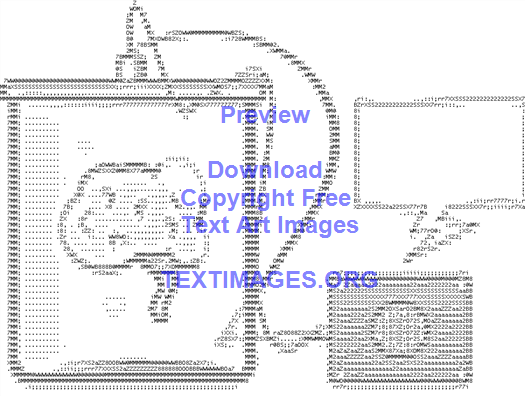"Displayed in the image is an intricate piece of ASCII art, a form of old-school digital art crafted entirely from keyboard characters such as letters, numbers, and symbols. This gray-toned illustration features a clear glass jar with a brain-like object floating inside. Extending from the jar are wires connected to what resembles a small speaker or an electrical box. Above the speaker, there’s a square text bubble, although it's empty. The detailed arrangement of lighter and darker text characters creates a textured, cartoon-like visual. Additionally, a watermark overlays the artwork, promoting textimages.org, where one can download copyright-free text art images."